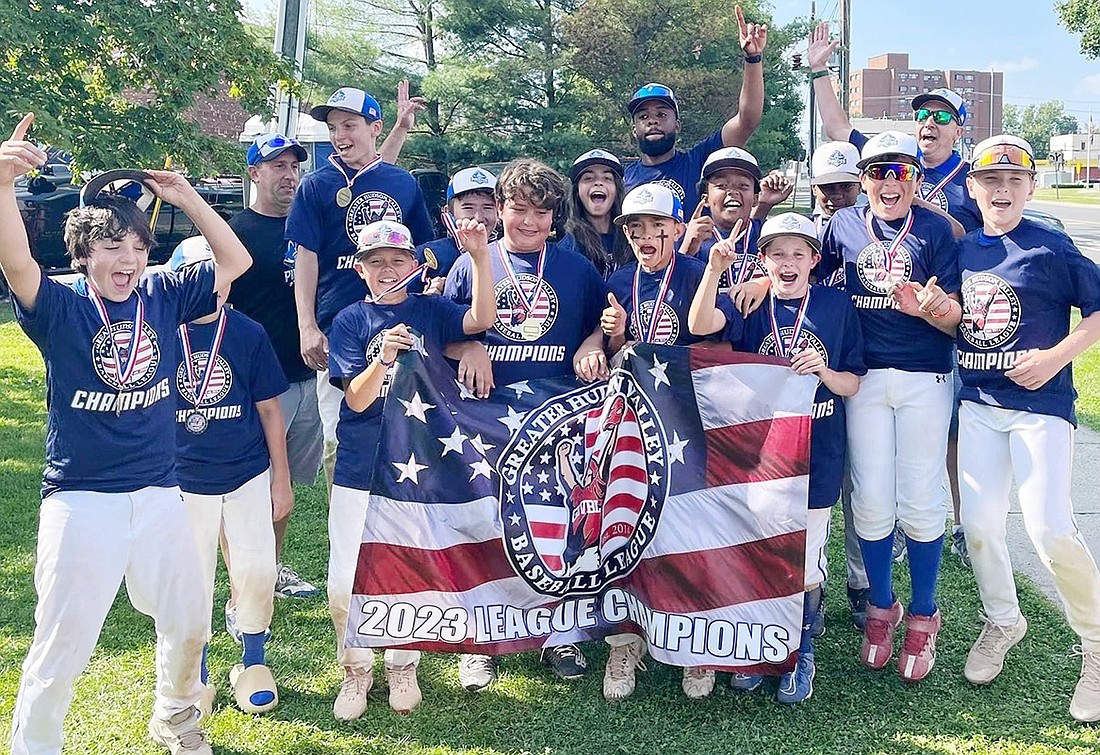This vivid photograph captures the jubilant moment of a youth baseball team celebrating their triumph as the 2023 Greater Huron Valley Baseball League Champions. Approximately a dozen to fifteen boys, aged around 10 to 15, occupy the foreground, all wearing blue shirts emblazoned with a red, white, and blue logo featuring an American flag and a baseball player with both arms raised. The word "Champions" is prominently displayed on their shirts. With baseball caps, white pants, and medallions hanging on red, white, and blue lanyards, the boys are beaming with joy, their hands raised in various gestures of victory—thumbs up, peace signs, and number one signs. They proudly hold a flag at waist height, which mirrors the emblem on their shirts and reads "Greater Huron Valley Baseball League 2023 League Champions." 

Behind the boys stand several adult men, presumably coaches, also caught in the exuberant moment, echoing the celebratory gestures. Their surroundings suggest a grassy park within a city, with a visible sidewalk to the right and a backdrop of trees and a red brick, ten-story apartment building in the top right corner. This detailed snapshot beautifully encapsulates the triumphant spirit and unity of the team.